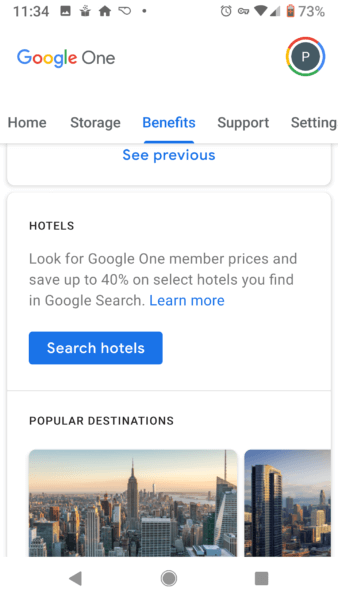This is a screenshot from a mobile phone with a white background. At the top-left corner, it indicates the time "11:34" in gray font. Next to the time, there are small icons for a photo, a house, and an alarm clock. The top-right section shows full Wi-Fi signal, two out of four bars of mobile signal, and a battery icon indicating 73% remaining.

Below these status icons, the screen displays the Google One app. The header shows "Google One" with a colorful circle to its right, featuring a gray circle within it and a white "P" in the center. Directly beneath the header, there is a navigation menu with the options: Home, Storage, Benefits, Support, and Settings, with the Benefits section currently selected.

A blue link labeled "See Previous" appears below the menu, followed by black text that reads "Hotels: Look for Google One member prices and save up to 40% on select hotels you find in Google Search. Learn more." Below this text, there is a prominent blue button with "Search Hotels" written in white font.

Furthermore, the screen displays the heading "Popular Destinations" in black font, under which two photos of the New York City skyline are featured.